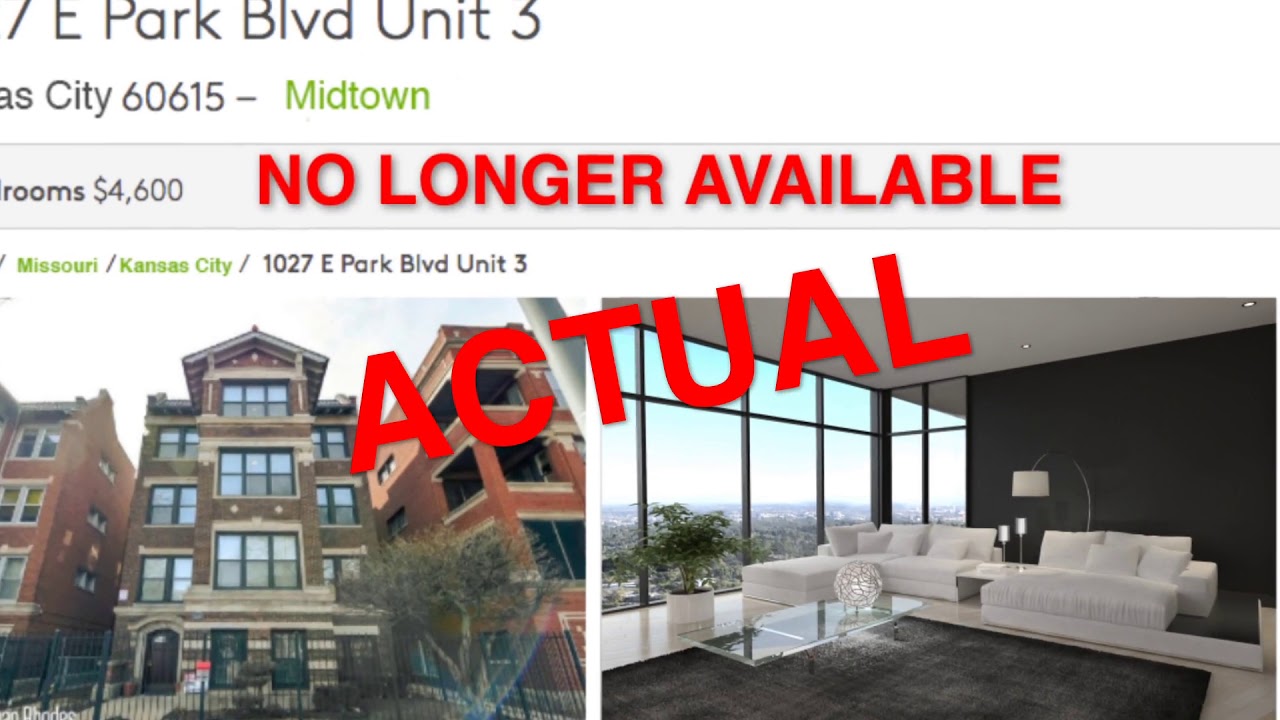Here is the cleaned-up and detailed caption for the image:

---

This image appears to be a partial screenshot taken from a website, likely using the snipping tool on Windows, capturing a panoramic view of a real estate listing.

At the top, partially cut off, black text reads: "7E Park Book BLVD 3." Additionally, in a section cut off at the top, it mentions "AS City 60615" in black letters, but with visible green text next to stating "Midtown." This suggests that the property is located in Kansas City, as the 60615 zip code prefix typically corresponds to that region.

Below this header, the caption is a gray text bar reading "rooms $4,600" in black letters, with a bold, all-caps notice in red letters stating: "NO LONGER AVAILABLE."

Further down, the caption includes additional information in green letters: "Missouri / Kansas City / 1027 E Park BLVD Unit 3." This confirms the location and unit details.

The image features two photographs of the place:

1. The left image shows the exterior of a brown building with large windows ascending to a pointed roof. Adjacent to it are several red-brick buildings. There is a black fence in front and a small tree to the right of the building.
2. The right image presents an interior view from the top of the building. The setting includes a large window offering a picturesque view, white sofas, a glass table, black walls, and a white ceiling.

Diagonal red text across the bottom of both images reads: "ACTUAL," likely indicating these are genuine photographs of the property.